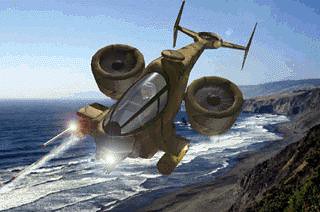The image depicts a detailed, full-color painting of a futuristic flying machine, resembling a hybrid between a helicopter and an airplane, soaring over a coastal landscape. The sky dominates the upper half with varying shades of blue, indicating a clear, sunny day. Below, the middle left displays a vast, turbulent ocean with waves crashing against the shoreline, transitioning from deep blue to white foam as they meet the rocky coast. The lower left section features rugged, rocky hills with a hint of greenery, possibly bushes or small trees, interspersed among them. 

Central to the scene is the tan or rustic-colored flying vehicle, which seems ancient or out of place compared to modern aircraft. It features downward-pointing motors, indicating a unique design, and is illuminated by lights underneath. The vehicle engages in some form of activity, emitting an undefined stream from its front. The cockpit reveals a helmeted pilot, adding a dynamic human element to the scene. The right side transitions to a sandy shoreline mixed with more rocky terrain and sparse vegetation. Overall, the image captures a vivid and imaginative outdoor scene filled with elements of nature and futuristic technology intertwined seamlessly.